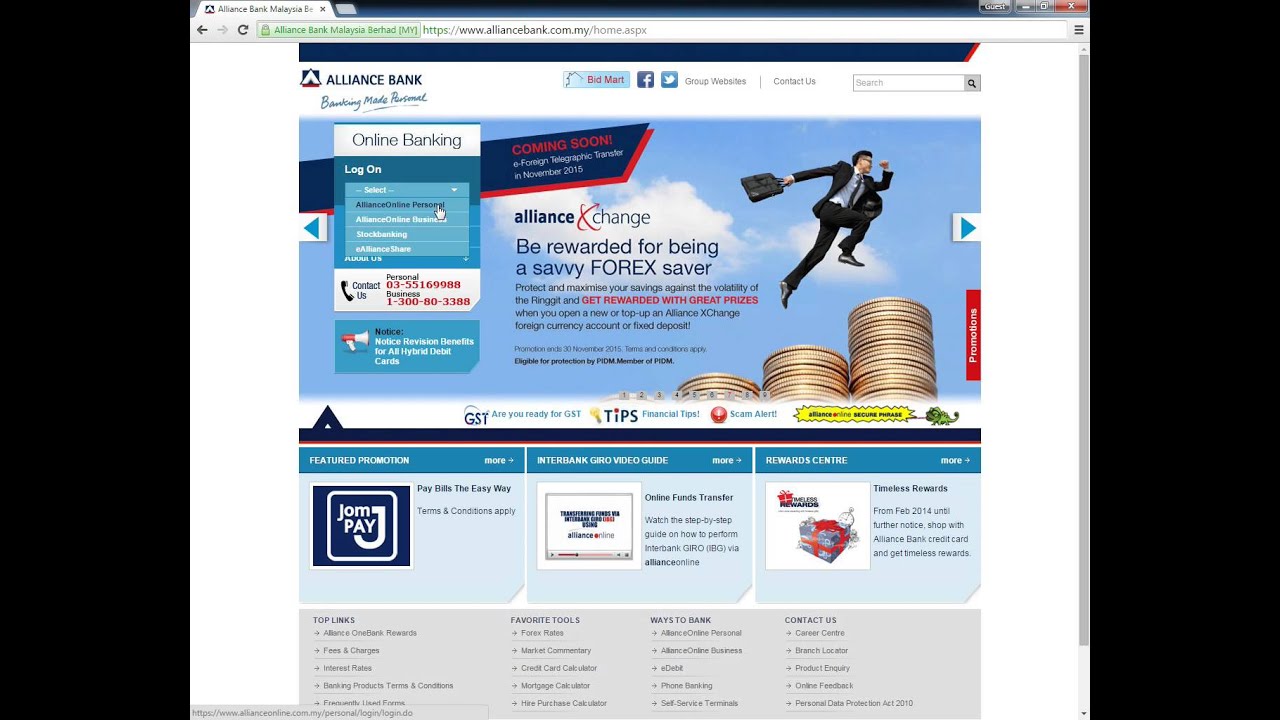This image showcases a detailed screenshot of the Alliance Bank Malaysia website, displayed in landscape mode. The top portion of the screen features two broad black strips running horizontally along the upper and lower sections of the image. In the upper left-hand corner, a browser tab is open, displaying the Alliance Bank Malaysia logo. On the upper right-hand corner, there's a "Guest" label followed by options to minimize the window and a red "X" button to close it.

Beneath this, the URL bar indicates a secure connection to "alliancebank.com.my/home." Following that, a prominent blue stripe stretches across the screen, with the Alliance Bank logo situated in the upper left-hand corner. Adjacent to this logo, possibly an advertisement for BidMart is visible. Just below this section are icons for social media links to Facebook and Twitter, as well as links to group websites and a "Contact Us" option. A search bar is also present for user convenience.

Directly under the logo, the text "Banking made personal" adds a welcoming touch. The focal point of the page is a large image depicting a man energetically jumping over money, accompanied by the tagline "Be rewarded for being a savvy Forex saver" under the "Alliance change" campaign. Below this image is a column listing various offerings including "Featured Promotion," "Interbank Video Guide," and "Reward Center," hinting that the website provides a range of services and promotional content related to banking and financial management. This screenshot captures the essence of a sophisticated and user-friendly online banking platform.